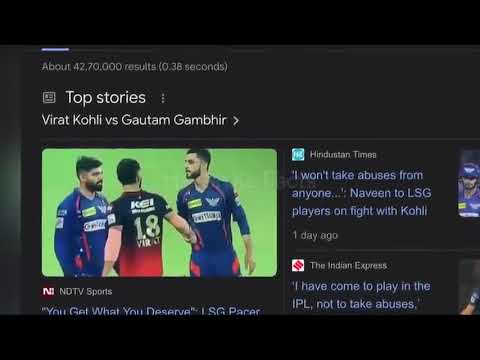The screenshot captures a section of a dark-themed web page showing search results, likely from a news website. At the top, it indicates approximately 42,070,000 results in 0.38 seconds. Below that is the heading "Top Stories" with a subheading "Virat Kohli vs. Gautam Gambhir." The image centered on the page features three athletes on green grass: two in blue uniforms and one in a red and black uniform, shaking hands. The man in the middle, donning the number 18 and salmon-colored elbow pads, faces the two in blue. On the right of the image are summaries of related articles: one from the Hindustan Times with the headline "I won't take abuses from anyone," and another from the Indian Express stating "I have come to play in the IPL, not to take abuses." Above the image, the page notes "NDTV Sports," followed by a quote "You get what you deserve SG Pacer." Related stories appear to the right of the image, emphasizing the ongoing narrative around the confrontation between Kohli and Gambhir.